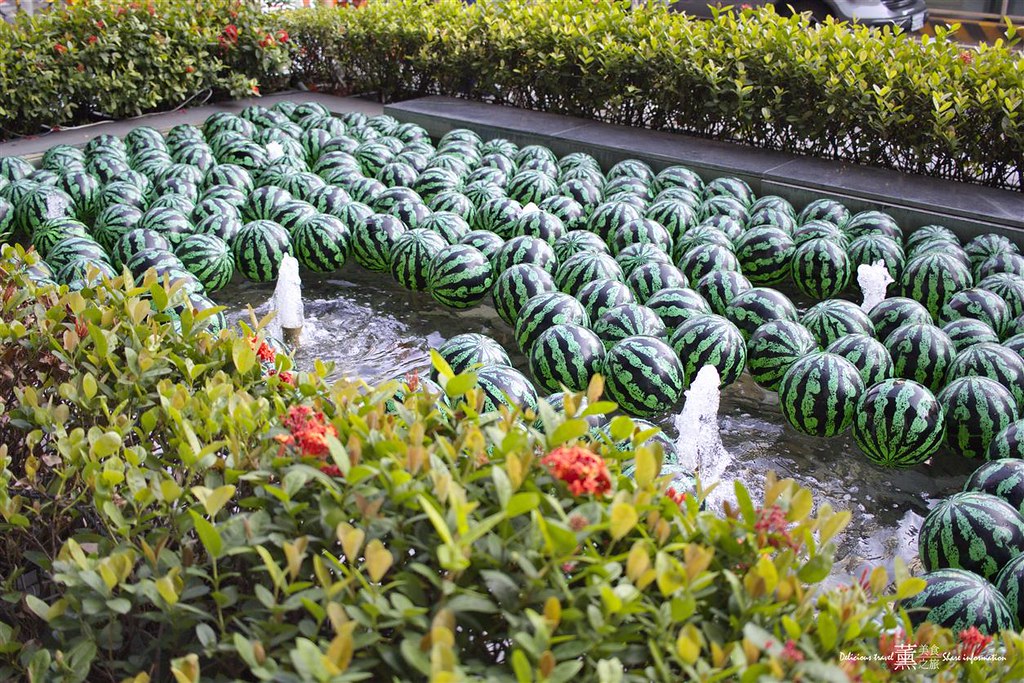The photograph depicts a charming garden featuring a square-shaped fountain encircled by manicured hedges. The fountain boasts three spouts, each gracefully shooting water into the air. The fountain's basin is filled with rubber balls imitating watermelons, their green and white patterns covering almost the entire water surface. Marble benches provide seating around the fountain, inviting visitors to sit and enjoy the serene surroundings. The garden also includes colorful flower arrangements, with clusters of red flowers and green plants adorned with pretty pink blooms. These vibrant plants are interspersed along the hedges, which display a gradient of green shades with lighter yellow tips. The entire composition creates a picturesque and whimsical atmosphere, blending natural beauty with playful elements.